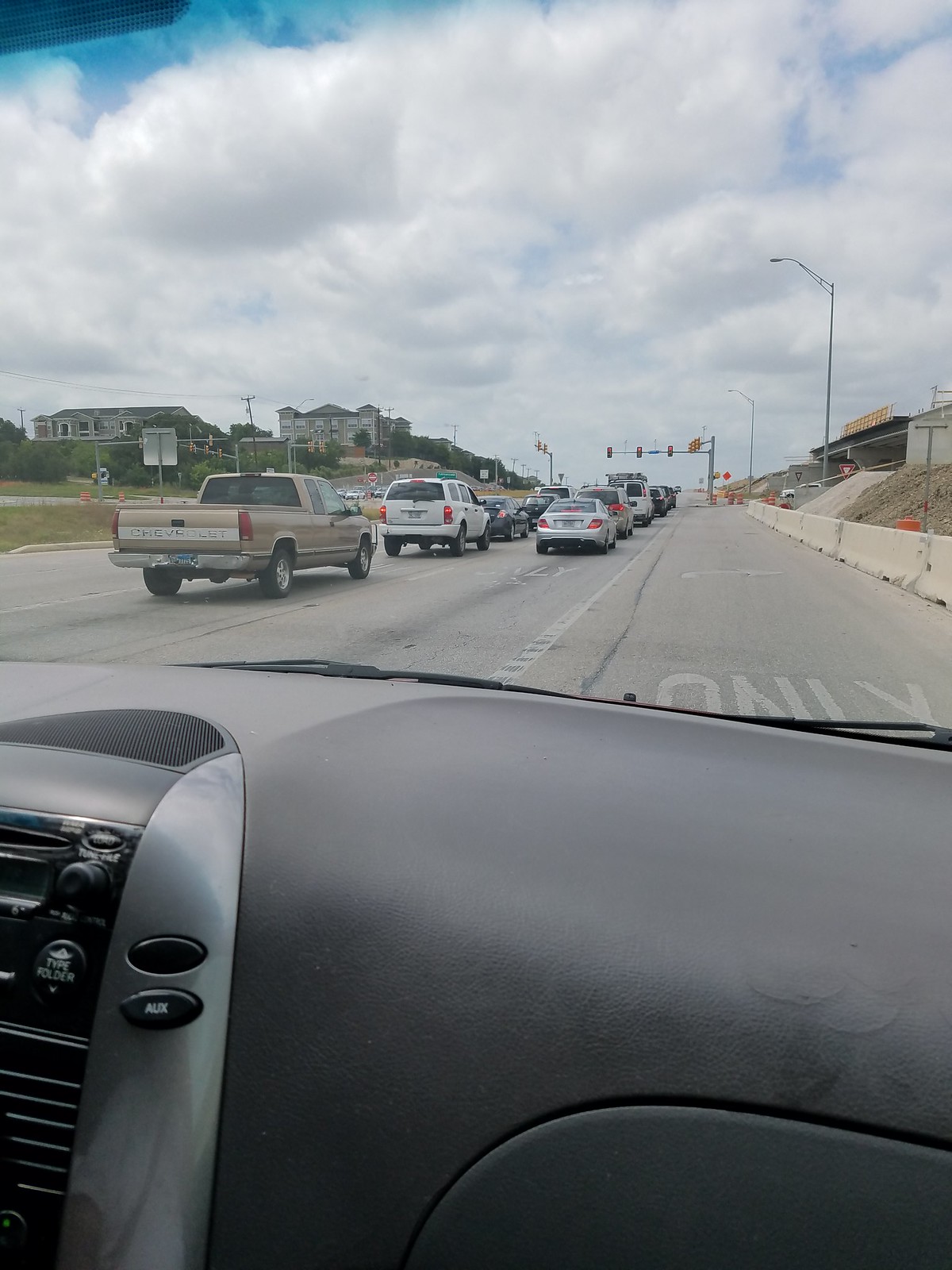The outdoor color photograph, taken in bright daylight from the inside of an American car's passenger side, looks through the windshield showing a gray dashboard with a metallic or chrome trim around the radio controls, including an AUX button. The car is either merging onto or parked in a "right-turn only" lane, as indicated by the partially visible painted word "ONLY" on the grayish road surface. In the lower part of the image, you see dash and console elements. The view through the windshield reveals traffic with vehicles in two lanes moving from the right to the center foreground, awaiting a traffic light just right of center in the background. In detail, these vehicles include a pickup truck, a white SUV, a black sedan, a possibly white van or truck, a silver sedan, a silverish minivan, a white truck with a ladder, and another black car. The scene is framed by concrete barriers with nearby dirt on the upper right and what appears to be bridge construction. To the upper left, a two-story gray building with a dark gray roof, possibly an apartment complex, can be seen amid a mostly cloudy, white sky.